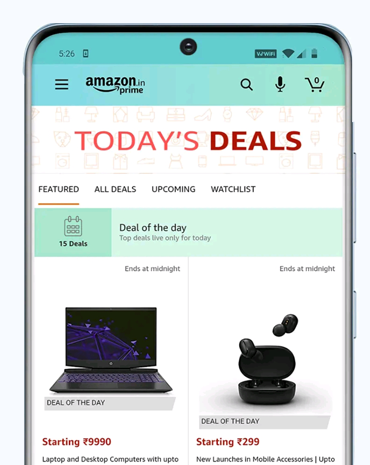The image appears to be an advertisement showcasing a smartphone screen that displays Amazon Prime deals. The time shown at the top left corner of the screen is 5:26, and various status icons such as the battery level, Wi-Fi, and wireless signal are visible on the right side. The header of the screen features a light turquoise border, slightly lighter than the background, and prominently displays the Amazon India logo ("Amazon.in"), with "Prime" written beneath it.

The main section of the screen has a white background with large, colorful text describing the deals. In bold pink font, it says "TODAY'S," followed by "DEALS" in a maroon font. Below this title, there is a navigation bar in gray font listing categories: "Featured," "All Deals," "Upcoming," and "Watchlist." 

A rectangular banner labeled "Deal of the Day" spans the width of the screen. Just below the banner, the deal itself is depicted with two primary products. On the left, there is a sleek black laptop with a purple keyboard, and its screen displays an image that resembles a purple flying saucer against a dark background. On the right, a black carrying case for wireless earbuds is open to reveal the earbuds inside.

The overall design and layout of the image strongly suggest that this is an advertisement, specifically targeting Amazon Prime users in India, and highlights a special deal of the day.